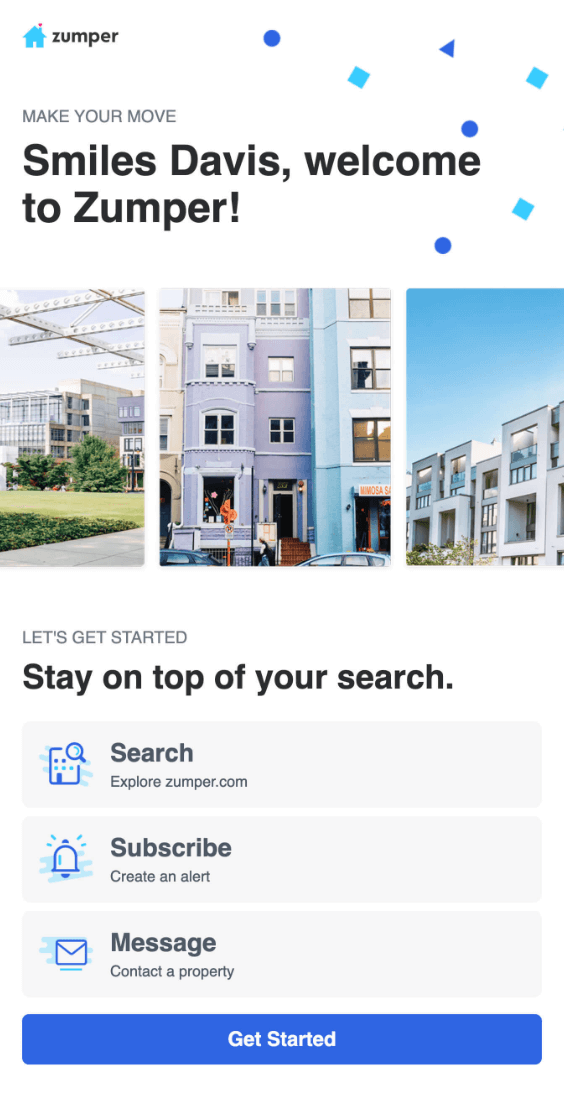The image depicts a mobile website screenshot from the company Zumper, identifiable by its vertical layout and modern, contemporary design. The interface prominently features a welcoming message: "Make Your Move, Smiles Davis. Welcome to Zumper." The screen showcases three images of various types of housing, indicating that Zumper facilitates property searches, similar to platforms like Zillow.

Below the introductory message, the user can find options to begin their property search and stay on top of their housing needs. These options include:
1. **Search** - Explore properties on zumper.com.
2. **Subscribe** - Create alerts for new listings.
3. **Message** - Contact property managers directly.

At the bottom, a noticeable bright blue button labeled "Get Started" suggests that users can unlock the features of searching, subscribing, and messaging by initiating their journey with Zumper. The overall aesthetic of the site is clean and minimalist, utilizing a color scheme of whites, blues, and grays to create a sleek and user-friendly interface.